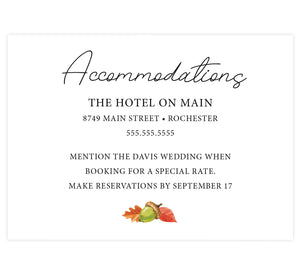The image depicts a white business card, seemingly intended for inclusion in wedding invitations to guide guests on accommodations. At the top center, "Accommodations" is elegantly scripted in black cursive. Below, the card provides key details in computer-printed black text. Prominently, it lists "THE HOTEL ON MAIN" in all capital letters, followed by the address "8749 Main Street, Rochester." The contact number "555-555-5555" is displayed beneath. A space separates this from the next section, which instructs guests to "Mention the Davis wedding when booking for a special rate," and advises, "Make reservations by September 17th." This text is centrally aligned. At the bottom, a colorful illustration features a green acorn with a yellow cap, flanked by two leaves: a red, bulb-shaped one on the right, and an orange, jagged-edged one on the left, adding a touch of autumnal charm to the card.